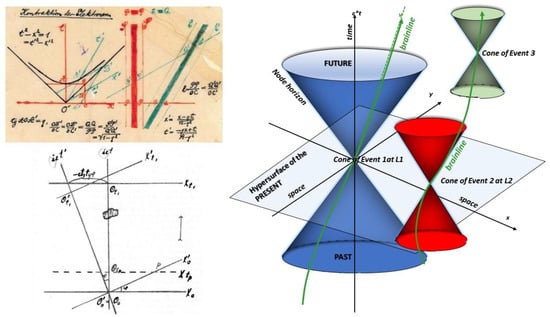The image contains three detailed diagrams, likely depicting scientific or mathematical concepts. Situated on the left side, the top left diagram is a geometrical illustration on a beige background, featuring a 90-degree angle marked with red lines. Below it, another geometrical diagram consists of a cross shape, a T-intersection, and a right-angle triangle pointing downwards. Dominating the right side is a larger, colorful scientific diagram labeled "hypersurface of the present" that includes mirror images of cones. Three sets of cones are depicted: a large blue cone (event 1), a large red cone (event 2), and a small green cone (event 3). These cones are interconnected by lines representing time, with the top labeled "future" and the bottom labeled "past." The overall impression is of educational content related to physics or metaphysics.